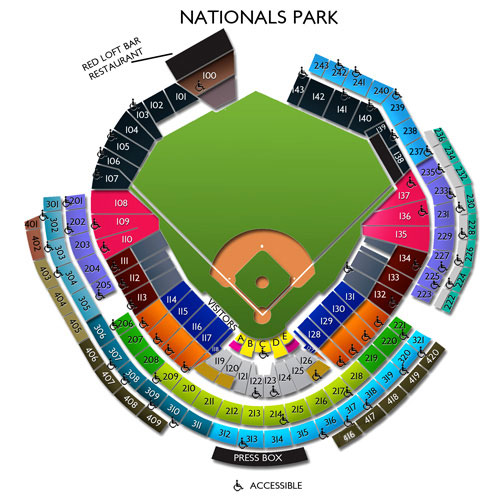The image is an intricate seat map of Nationals Park, a baseball stadium. Dominating the center is the detailed baseball diamond, featuring a lush green outfield contrasted with a brown infield. The catcher's plate and the pitcher's mound are highlighted in brown, with the bases marked in white, extending along the foul lines. The seating arrangement radiates outward from this central field. On the right edge of the field, the home team seats are depicted in white, while the visitor's seats are designated along the left edge, labeled in black and white.

In the top left corner of the stadium map, the "Red Loft Bar-Restaurant" is noted, positioned past the center field area. This section includes dark blue seats, with lighter blue seats situated further back to the right, forming a semi-circular shape. The bottom section of the map features a black-inked press box, identified with a "press" label. Directly underneath, there is a section marked as "accessible," accompanied by a handicap sign, indicating the availability of seats for guests with disabilities.

The seats directly behind home plate stand out in yellow, flanked by pink seats on either side. This comprehensive overview captures the varied seating options and key locations within Nationals Park, providing a clear understanding of the stadium's layout.